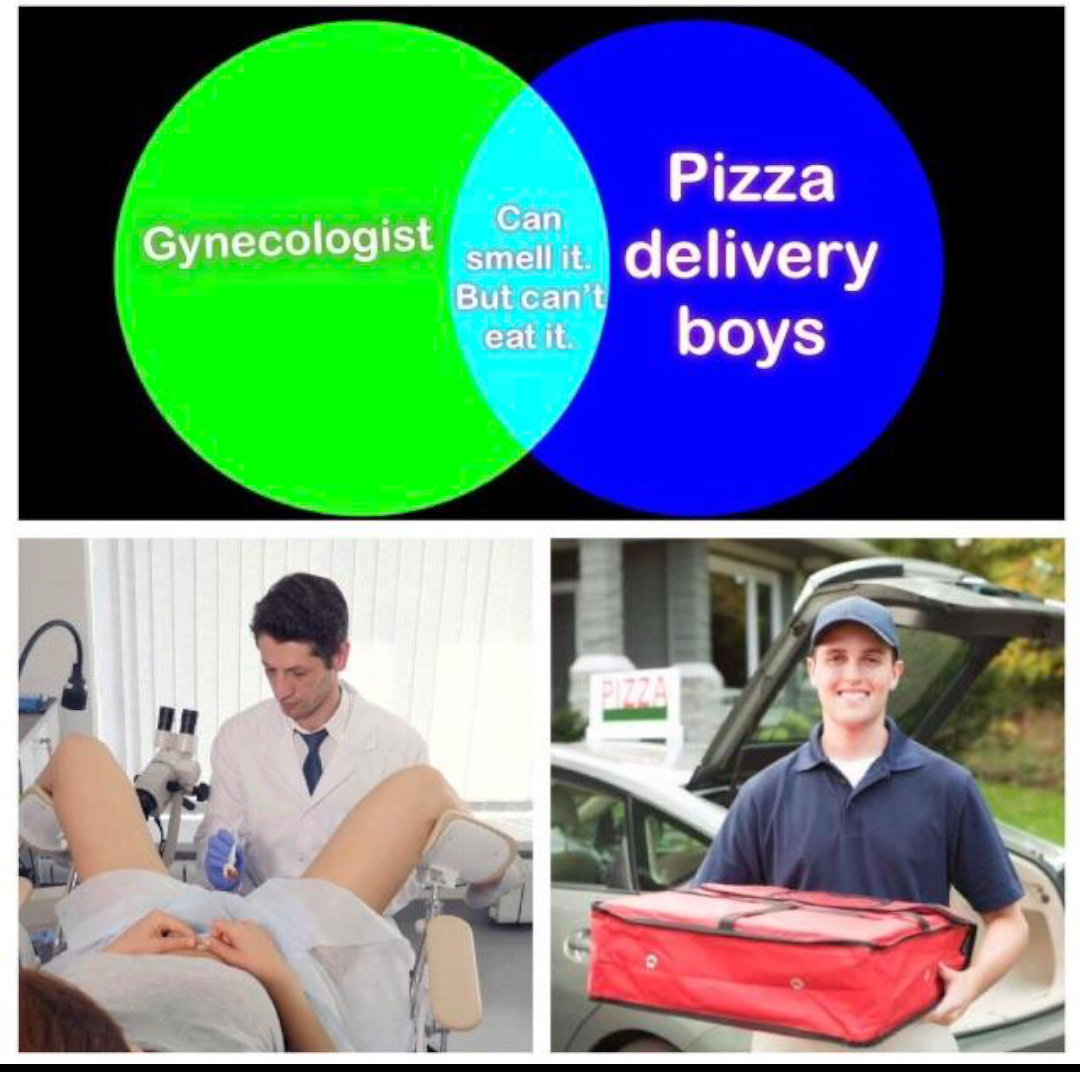The image is a meme, and it's structured into three sections. At the top, there's a Venn diagram with overlapping circles. The left circle is green and labeled "Gynecologist," while the right circle is blue and labeled "Pizza Delivery Boys." The overlapping section in the center is light blue and contains the text "Can smell it, but can't eat it."

Below this diagram, the image divides into two parts. On the left, there's a clinical scene featuring a gynecologist performing a vaginal examination with a woman in a robe lying in stirrups. The gynecologist is wearing a full medical outfit, including gloves. On the right, there's an illustration of a pizza delivery boy wearing a navy blue baseball cap and t-shirt, standing by his car with a red pizza bag. The car has a visible pizza sign on the roof, and behind it is a house.

The image features various colors, including black, green, light blue, dark blue, pinkish white, red, and gray. The overall setup and style suggest it is designed to be a meme shared online.